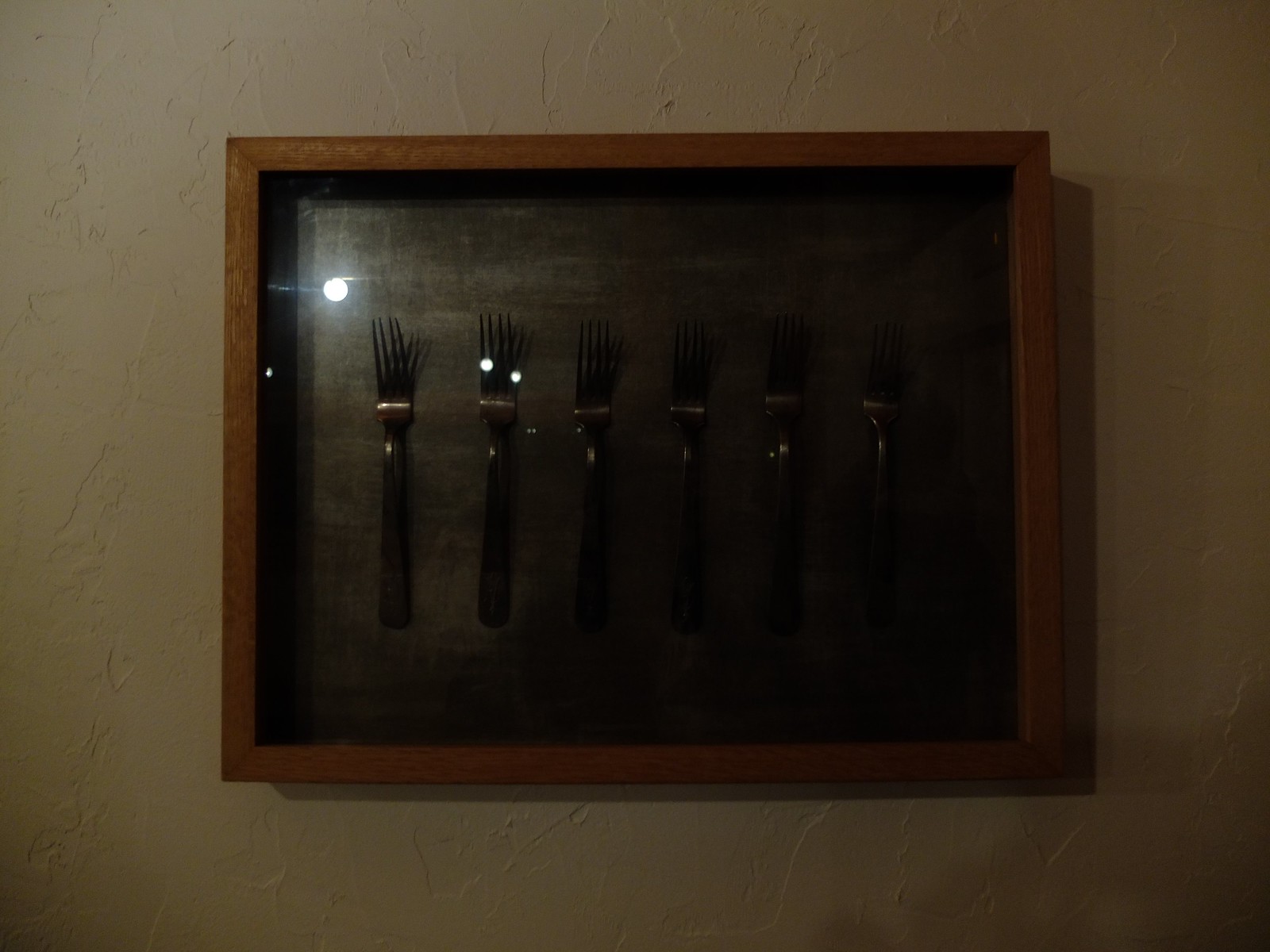This photograph captures a framed piece of art hanging on a dark gray, slightly brown-hued plaster wall. The medium brown wooden frame encloses a display case with a black, wood-textured background. Inside the frame are six forks arranged side by side, presented as an art piece. The glass covering the display reflects a bright light in the top left-hand corner, partially obscuring the view and casting a glare over the image. The wall behind the frame is dimly lit, emphasizing the dark tones of the artwork and the unusual presentation of the cutlery.